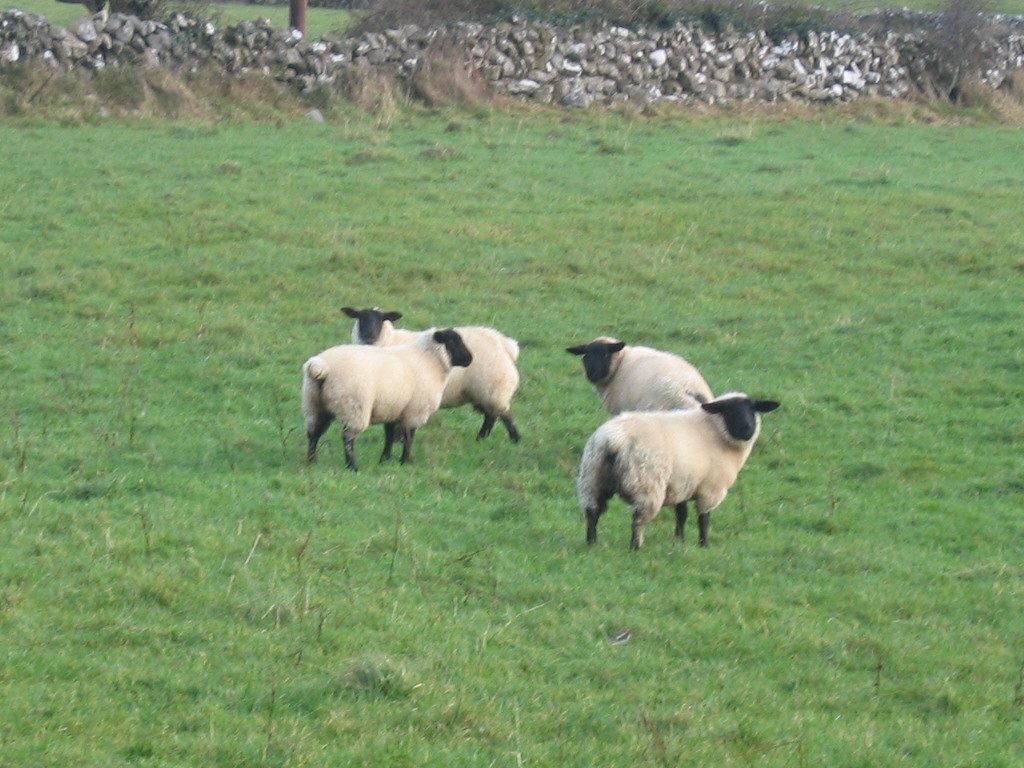In the foreground of this image, a vast green pasture stretches across nine-tenths of the frame, its verdant grass appearing well-nourished but slightly uneven in height. Occupying the center of this pasture are four notably long-haired sheep, poised to be sheared. These sheep are distinct with their contrasting black faces, ears, legs, and tails against their white fluffy coats.

Three of the sheep gaze directly into the camera with their featureless black faces, while the fourth sheep looks to the right. Their arrangement places two sheep closer together on one side and another pair on the opposite side, each displayed in varying angles of profile. The grass around them, not freshly mowed, shows clumps of taller blades and scattered twigs.

In the distant background, the remaining top one-tenth of the image features a rocky structure, possibly a crumbling stone wall or a fence made of boulders and gravel. This barrier separates the immediate pasture from another field glimpsed further back. On the top-left corner, a solitary fence post stands out against this rustic backdrop, emphasizing the rural setting.